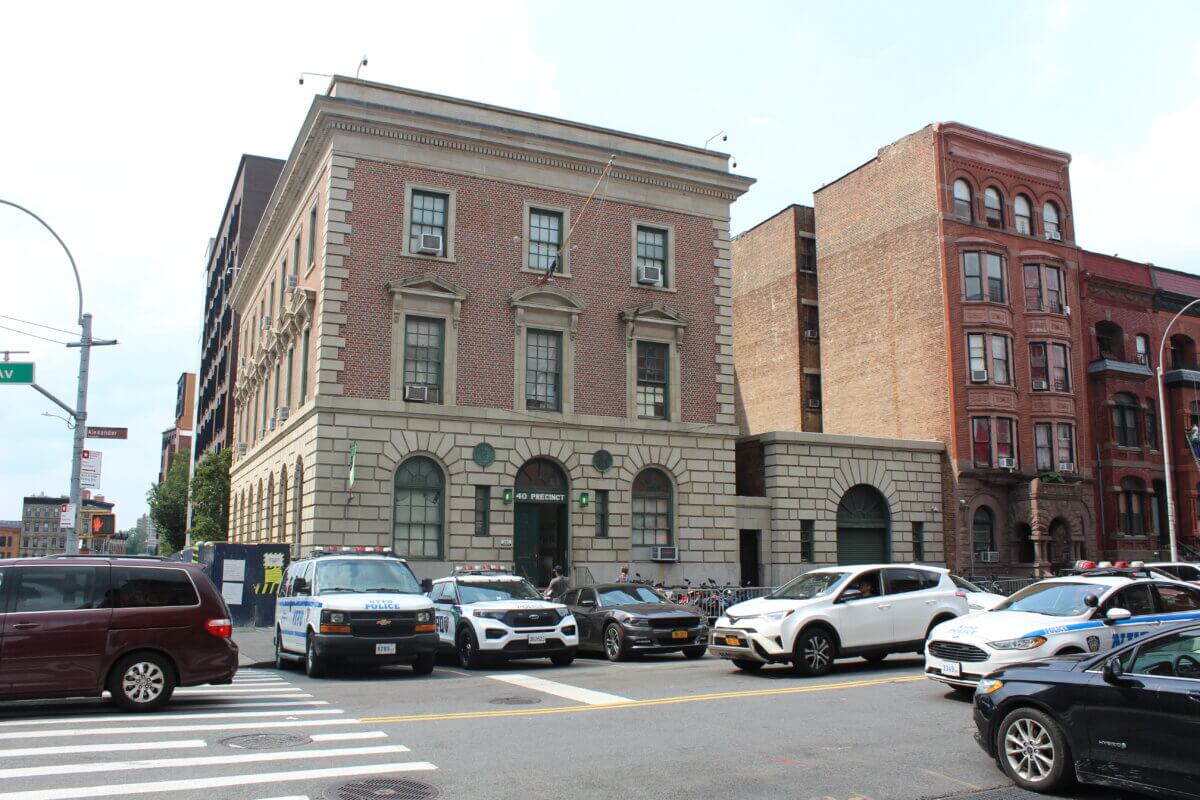This photograph captures a bustling city block dominated by a three-story brick police station marked as the Fourth Precinct, identifiable by the sign on its facade. The architecture hints at an older design, evident through the two window-mounted air conditioning units. The police station stands on the left side of the image, flanked by other brick buildings, one resembling an apartment complex with ten windows and classic red bricks. The central precinct building itself exhibits a pattern of eight windows in a rectangular configuration and is constructed with mixed beige and red bricks.

In front of the police station, there are three marked police vehicles. Two of these are parked while the third is in motion, traveling towards the left side of the frame. A half-visible van is crossing the street, partially over a crosswalk towards the camera. Additionally, several motorcycles are parked behind a barricade near the precinct. The street scene is busy; several vehicles, including those in motion and others waiting at the traffic light, populate the frame. Among the moving cars, one appears to be turning into a lane bound for the left. Pedestrians are visible near the entrance of the police building, adding to the urban liveliness of the scene. The weather is clear, highlighting the intricate details of this active city street.